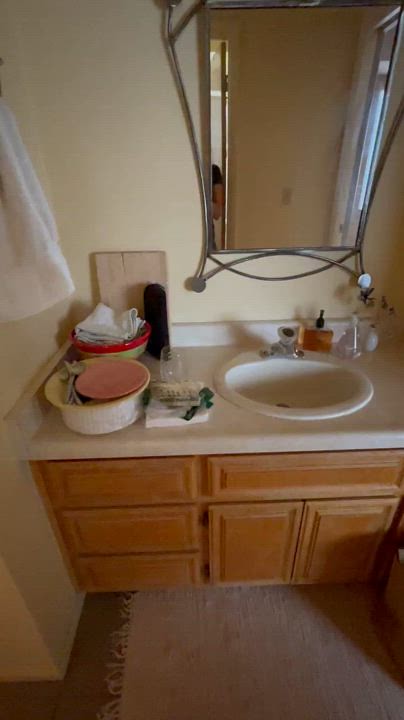A cozy washroom is depicted in this photo, featuring a pristine white rug centered on the floor. The walls surrounding the space are painted white, exuding a clean and calming atmosphere. Dominating the foreground is a set of elegant brown cabinets with two doors and three drawers, topped with a sleek white countertop. The countertop houses a modern white sink, flanked by bottles with pumps for easy access to toiletries.

To the left of the sink, various items are meticulously arranged on the counter, including a white object with black and gray accents, a stack of plates, and some neatly folded white cloths. Additionally, a board rests against the wall, adding a touch of homeliness. The left side of the washroom features a white towel hanging on the wall, ready for use.

Above the sink hangs a large mirror, framed with decorative metal rods on either side. The mirror reflects part of the washroom's layout, showing a wall, a door, and an adjacent doorway through which a person can be seen, identifiable by their black t-shirt and a portion of their arm, adding a subtle human presence to the scene.